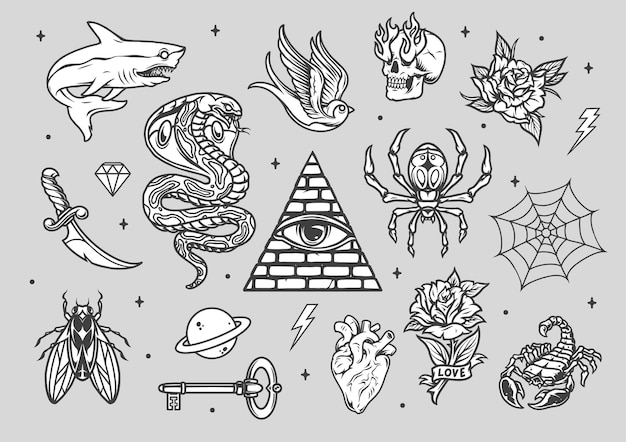The digital art piece is a horizontally aligned rectangular image with a solid light gray background, featuring an array of smaller black-and-white drawings arranged in a structured yet eclectic pattern. Starting from the top left and moving left to right, there is a shark, a bird, a skull with flames emanating from its eye sockets, a single flower with encompassing leaves, and a lightning bolt.

In the middle section, from left to right, there is a curved dagger, a small diamond, a large cobra snake, a pyramid with an eye at its center, a descending spider, and a spider web.

The bottom row, also from left to right, includes a fly viewed from above in an upward crawl, the planet Saturn, a key, a lightning bolt, an anatomically correct heart, another flower with the word "love" draped over its stem, and a scorpion. An eye within a pyramid with a brick pattern occupies the central position of the artwork. Scattered throughout the image are numerous little dots and plus signs, adding to the intricate detail of the piece.